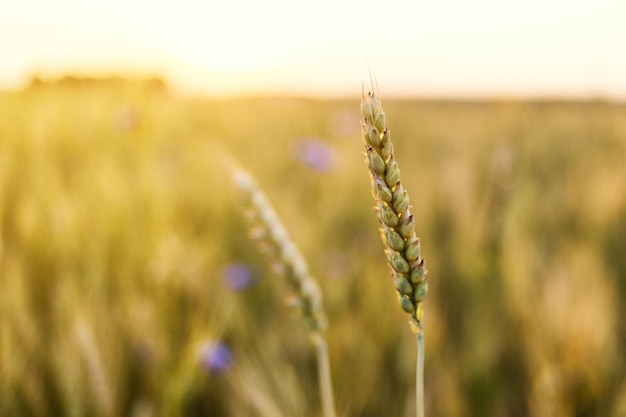The photograph depicts a serene field of wheat bathed in the warm hues of a setting sun, casting a golden glow across the scene. In the foreground, two wheat stalks dominate the composition. One stalk is prominently centered and in sharp focus, showcasing intricate details of its structure, with hues of yellow, green, and brown on its seed heads. Behind it, slightly blurred, is another stalk that stands out against the background. The field stretches into the distance, rendered in soft focus, creating a dreamy effect with yellow and purple tones suggesting scattered flowers and lens flares. The horizon is awash with bright oranges and yellows, indicating the sun's position just below the frame, enhancing the image's ethereal quality. Small, circular, transparent purple lens flares add a touch of mystique to the photograph, further enriching its atmospheric essence.